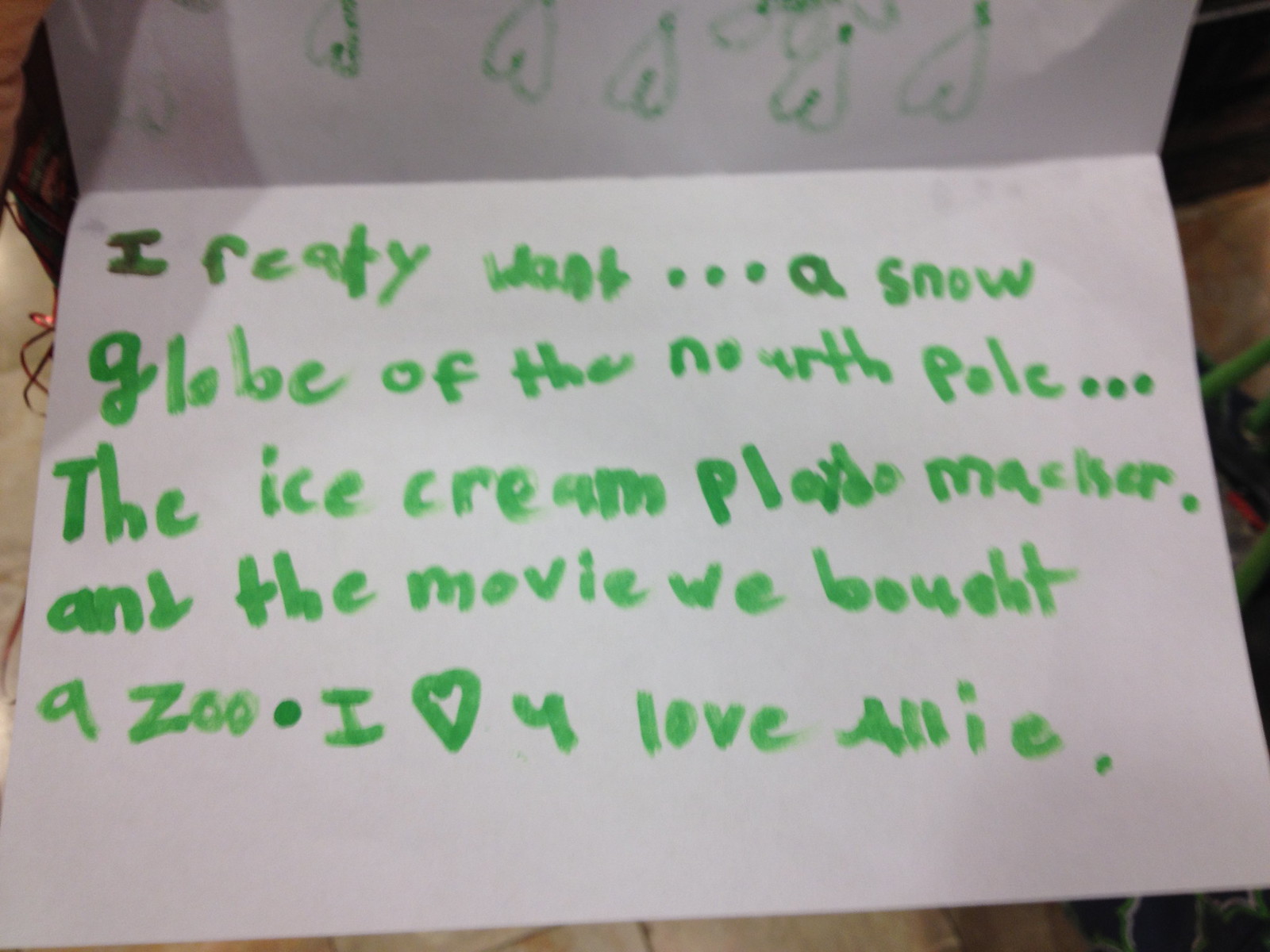This close-up photograph captures a child's handwritten note, likely a letter to Santa Claus, written in green marker on a white piece of paper folded in half "hamburger-style." At the center of the image, we see Allie's heartfelt message, marred by various spelling errors characteristic of childlike handwriting. The note reads, "I really want a snow globe of the North Pole, the ice cream Play-Doh maker, and the movie We Bought a Zoo. I heart you, love Allie," complete with misspellings like "Nourth" for North and a unique rendition of "really." Green hearts drawn by Allie are visible on the front, some bleeding through to the inside of the paper. Surrounding the note, indistinct objects on the border hint at a cozy indoor setting, possibly taken at night in a living room. The note, endearing and sincere, showcases the innocent wishes of a child.